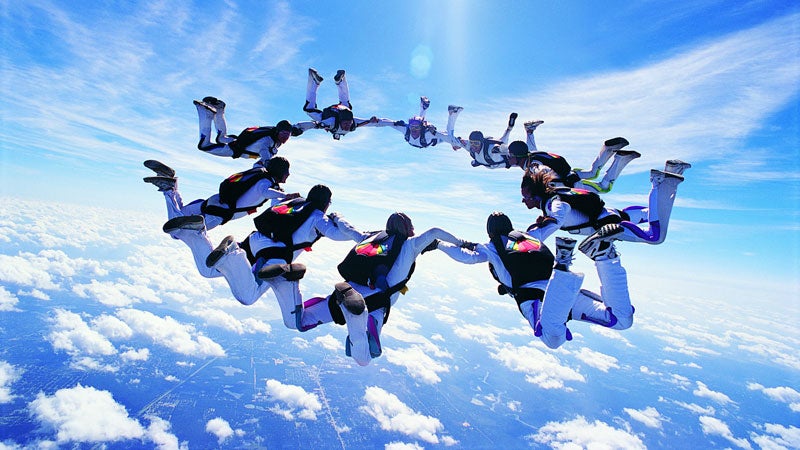This is a detailed photograph taken outdoors during the daytime, capturing a stunning mid-air scene with a group of skydivers. The rectangular color image, approximately six inches wide and three inches high, showcases the exhilarating moment from a clear vantage point, likely using a drone or GoPro camera, giving us a bird’s-eye view. We see about ten parachutists, all in matching white jumpsuits with black helmets and black parachute packs that feature vibrant red and blue or orange fabric details. The skydivers form a perfect circle, holding hands with their legs bent at the knees and feet elevated, facing each other in unison.

The upper half of the image is filled with a brilliant blue sky adorned with long, wispy white clouds, and beams of sunlight filtering down from the top center. The bottom half of the image transitions to fluffy, thick white clouds, beneath which the earth’s surface is just visible, displaying faint grid lines of roads, trails, and hints of city structures with trees and buildings. This captivating snapshot not only captures the skydivers’ synchronous formation but also the vast, beautiful backdrop of the serene sky and distant ground below.